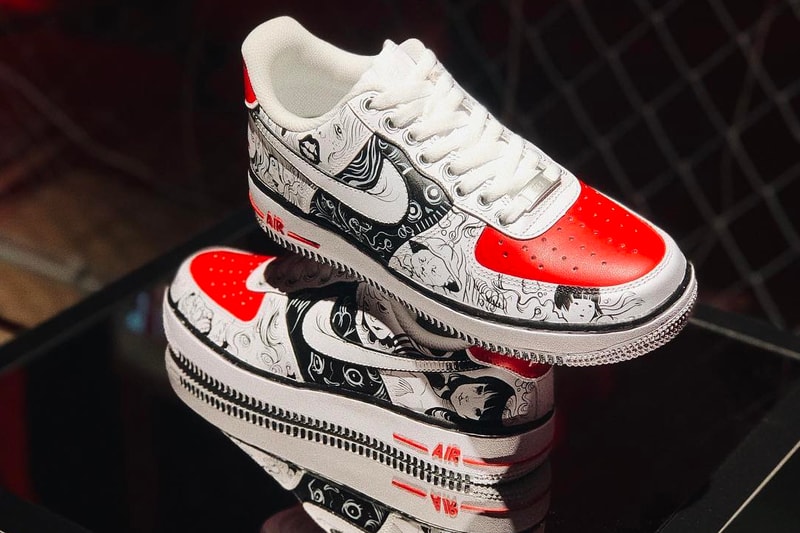The horizontally aligned rectangular image features a pair of Nike tennis shoes with a retro design, displayed on a reflective black surface. The shoes are positioned centrally, with the right sneaker resting atop the left sneaker. The toe of the upper shoe points towards the lower right corner, while the toe of the bottom shoe points towards the upper left. Predominantly white, the sneakers are adorned with intricate black and white cartoon and comic-style drawings, including characters such as a cat in a hat and various girls with different hair colors. The front and back parts of the shoes feature red accents, and the white Nike swoosh is prominently displayed. The soles of the shoes are white, marked with the word "AIR" in red, flanked by two red lines. The background includes a chain-link fence pattern in the upper right and a brown floor on the left, suggesting an outdoor setting.